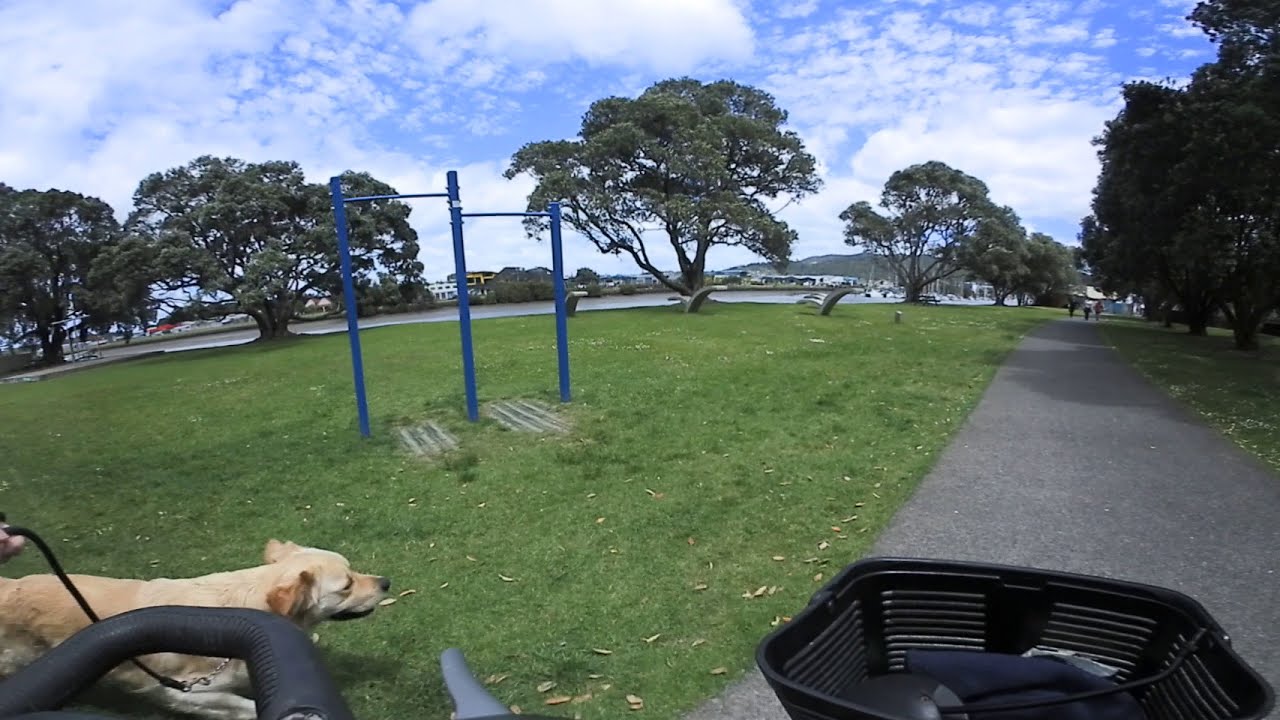In this photograph captured on a bright, sunny day in a public park, we see a scenic blend of nature and urban life. The bottom right corner features a black plastic basket, likely attached to a bicycle, suggesting the perspective of someone riding through the park. A handlebar is visible in the bottom left corner, and extending from it, a hand holds a black leash attached to a golden Labrador walking towards the right, nearly crossing the paved bike path that stretches from the foreground into the middle of the frame. 

To the left of this path, a large grassy area is adorned with several trees and intersected by blue metal posts designed for pull-up exercises. Beyond the grass, there's a river with a cityscape visible on the opposite bank. A bench is positioned on the grass, providing a perfect spot to take in the view. Above, the sky is a vivid blue, dotted with large, white puffy clouds, completing this picturesque outdoor scene.